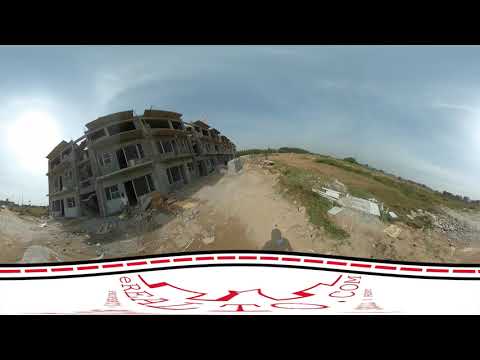This outdoor image appears to have been captured using a fisheye or VR lens, resulting in a slightly distorted, rounded view. Set during daytime, the sky above is predominantly blue with streaks of white and some gray clouds. The sun, nestled among the clouds on the left, casts light over the scene. 

The landscape features a dirt and rock hill with scattered patches of green grass and debris. Amidst this terrain stands a large, abandoned, and eroded structure with an undulating form that rises to three or four stories, following the hill’s uneven dip and rise. On the left, a person is walking along a dirt path that curves through the scene, marked by tan and brown hues. Their shadow is visible on the ground beneath them.

At the bottom of the image, a rectangular black frame partially encases a white, curvy line with red and black borders, which distorts the text "lto.com." Various details highlight the ruined and abandoned state of the buildings and the sparse, struggling vegetation spread across the area, enhancing the post-apocalyptic feel of the image.